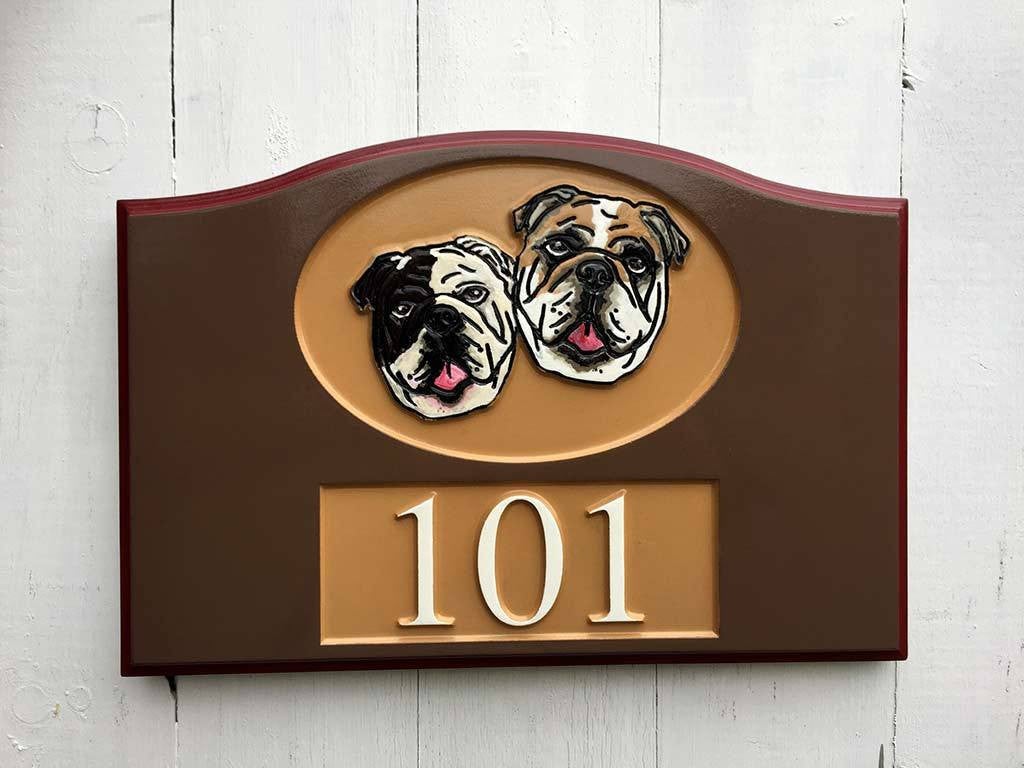This outdoor photograph captures a close-up of an aged house address sign mounted on a weathered white wooden wall with streaky paint and noticeable panel lines. The sign, which has a slightly arched top and square sides and bottom, features a bold red border along the arched section. Within the sign, a light brown oval at the top showcases detailed engravings of two bulldogs—on the left, a black and white bulldog, and on the right, a brown and white bulldog. Beneath the oval is a beige rectangular space with elegant white text that reads "101," denoting the house number. The plaque's background color is a solid brown, providing a stark contrast to the lighter engravings and the white text, making it easily readable and visually striking.